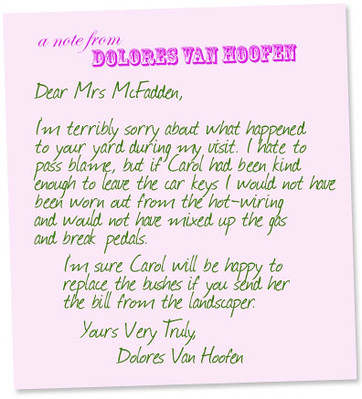The image shows a humorous note penned by Dolores Van Hoofen. Set against a soft pink paper background, the note introduces itself at the top with the phrase "A note from Dolores Van Hoofen" in bright, decorative purple typography. The body of the note is written in green and reads: "Dear Mrs. McFadden, I'm terribly sorry about what happened to your yard during my visit. I hate to pass blame, but if Carol had been kind enough to leave the car keys, I would not have been worn out from hot wiring and would not have mixed up the gas and brake pedals. I am sure Carol will be happy to replace the bushes if you send her the bill from the landscaper. Very truly yours, Dolores Van Hoofen." The text spans from the initial apology to offering a solution for replacing the damaged bushes, conveying a mix of humor and sincerity.